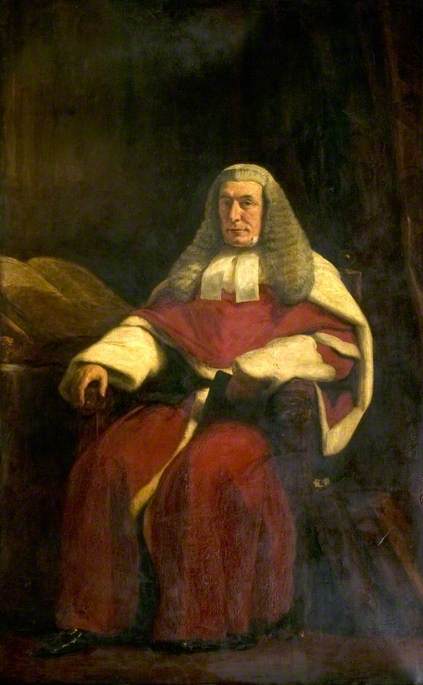This detailed, vertical portrait appears to be an old oil painting, possibly from the 1700s or 1800s, depicting a serious-looking, elderly white man seated in a wooden chair. The man is adorned in a red robe with voluminous white sleeves ending around the elbows, tied with a white cord. He also wears a white cape which adds a regal touch resembling a blend between a judge and a Santa Claus outfit. His long, wavy, grayish powdered wig frames his face in curls, reminiscent of historical fashion. The background is predominantly dark with a shadowy ambiance, accentuating an antique, aged feel. To his side, there is a table with an ancient, open book with yellowed pages. His black, shiny boots are visible, adding to his dignified appearance. The artwork shows signs of wear with some faded colors and white streaks at the bottom, indicating its historical value.